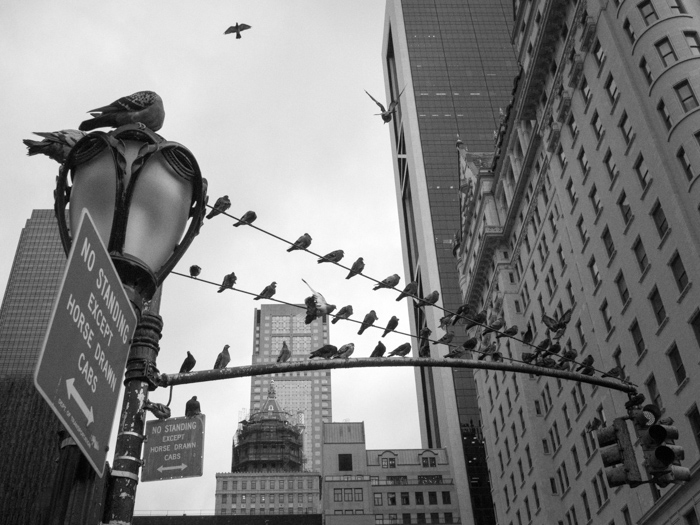This black-and-white photograph captures a nostalgic cityscape scene, likely in a major United States city like New York or Chicago. The image is viewed from the ground looking upward, prominently featuring a streetlight with an attached traffic signal. Multiple birds, possibly pigeons, are perched on the streetlight, its arm, and on three wires that extend diagonally from the left to the right, giving the impression that they "own" this part of the city.

On the left side of the image, a sign reads "No Standing Except Horse-Drawn Cabs," and an identical smaller sign is attached nearby, both frequented by birds. The right side of the photograph is dominated by tall buildings, including skyscrapers and other modern and less modern structures, set against a stark white sky. The overall composition evokes a sense of timeless urban life.